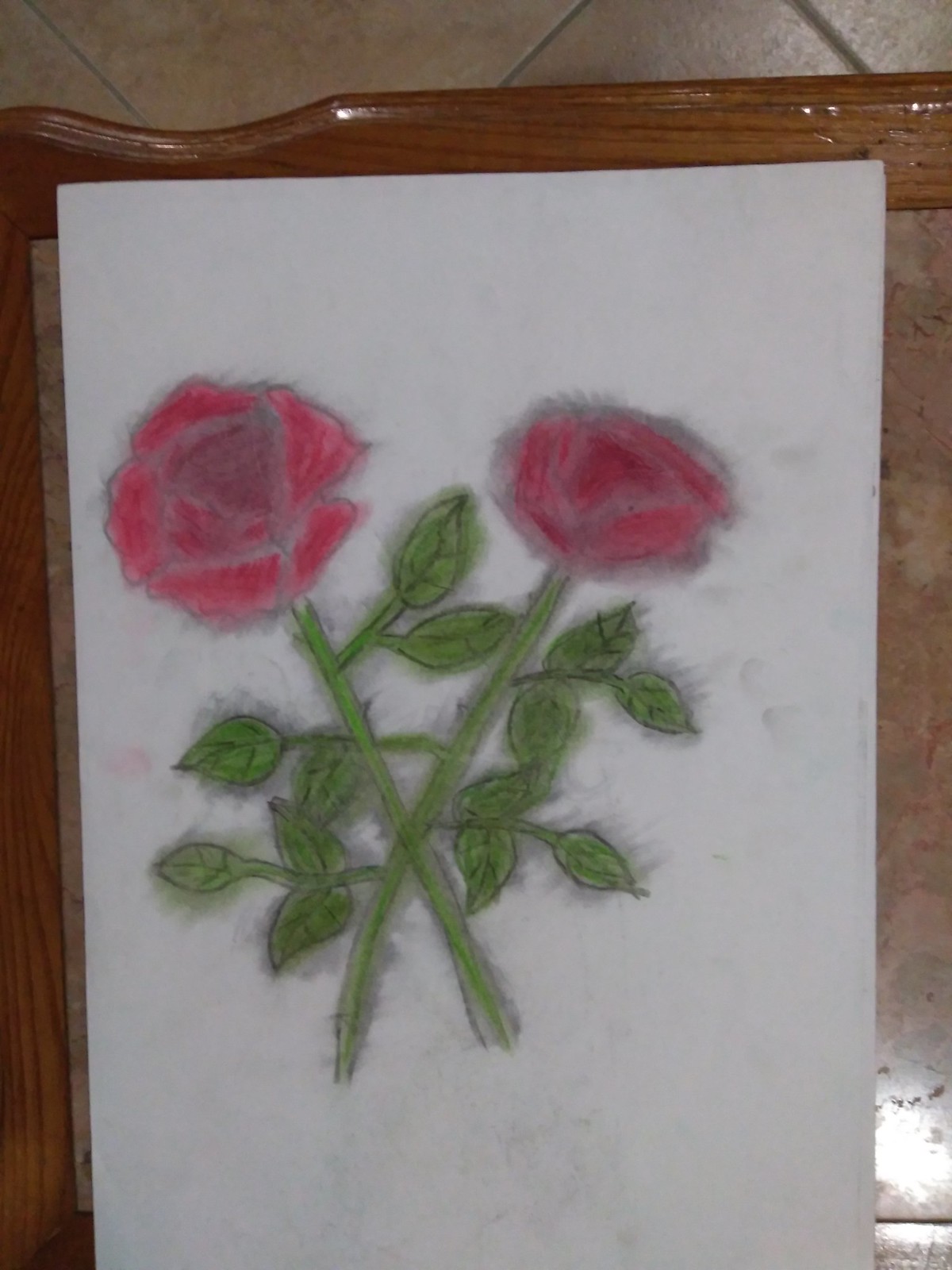The image showcases a hand-drawn illustration of two roses, crossing each other in an X shape, on a white A4 paper. Each rose is a vivid red or pink color, accented with detailed pencil outlines and colored pencil shading. The green stems are long and thin, intersected by multiple leaves, and the drawing employs deliberate smudge marks across the flowers, stems, and leaves, adding texture and an intentional artistic effect. The paper appears slightly smudged along the edges, enhancing the drawing's rustic charm. The sheet is lying flat on a brownish wooden table with shiny edges, positioned over a tiled floor with large off-white tiles and gray grout. The overall scene is photographed from above, capturing both the drawing and a glimpse of the surrounding environment.